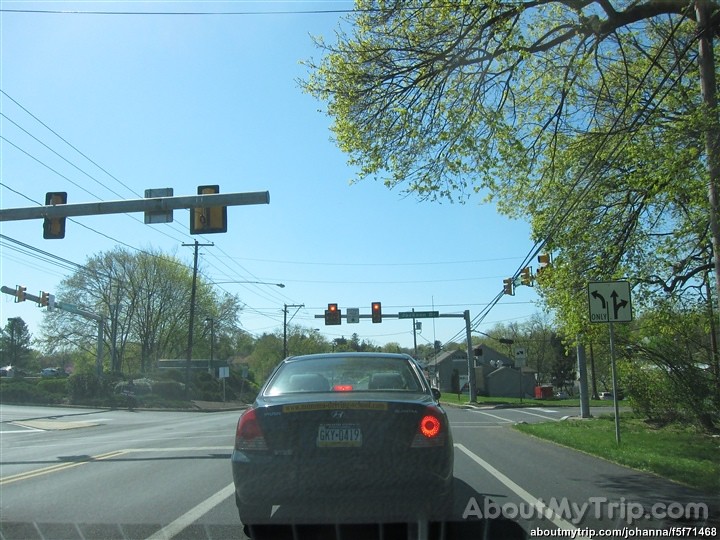In this image, a green Hyundai car with the license plate GKY0419 is stopped at an intersection, waiting for its turn to proceed. The car is centrally positioned in the frame. To the right of the image, abundant greenery including trees and foliage is visible, along with a traffic light pole and various electricity poles and wires extending across the scene. Attached to the traffic pole is a street sign indicating lane directions: left only, and straight or right. The background features what appears to be a residential neighborhood with at least two visible houses. On the left side, additional greenery and more street poles with electricity cables can be seen. The sky is clear and bright blue, suggesting fair weather. At the bottom right of the image, there is text promoting a website, mytrip.com, with smaller lettering below it that reads mytrip.com/Joanna/F5F71.